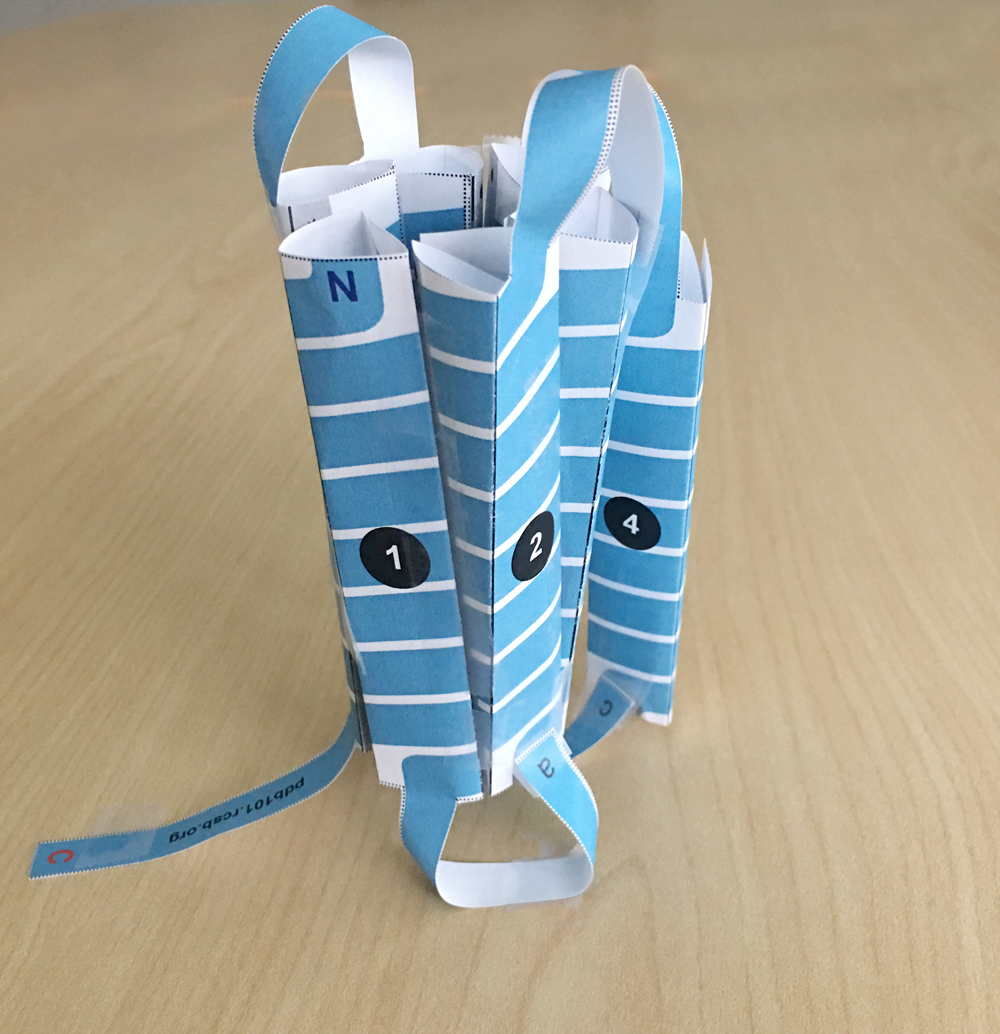In the image, we see various pieces of white paper, each meticulously folded into long, 3D triangular prisms. These prisms are connected by blue bands of paper, affixed with scotch tape, and are aligned upright on a wooden tabletop. The folded paper segments are arranged side by side, displaying numbers 1, 2, and 4 in white text within black circles. Additionally, a prominent blue letter 'N' is embossed on one of the blue bands at the top. The entire structure is reinforced with ribbon handles attached on both the top and bottom, and a big string can be seen coming out from the bottom. Horizontally, the white paper has blue stripes printed on it, and a specific strip bears the text "PDB101.RCSB.org" with a red 'C' at the bottom. It appears to be some form of intricate, possibly instructional or decorative assembly, although its exact purpose remains unclear.